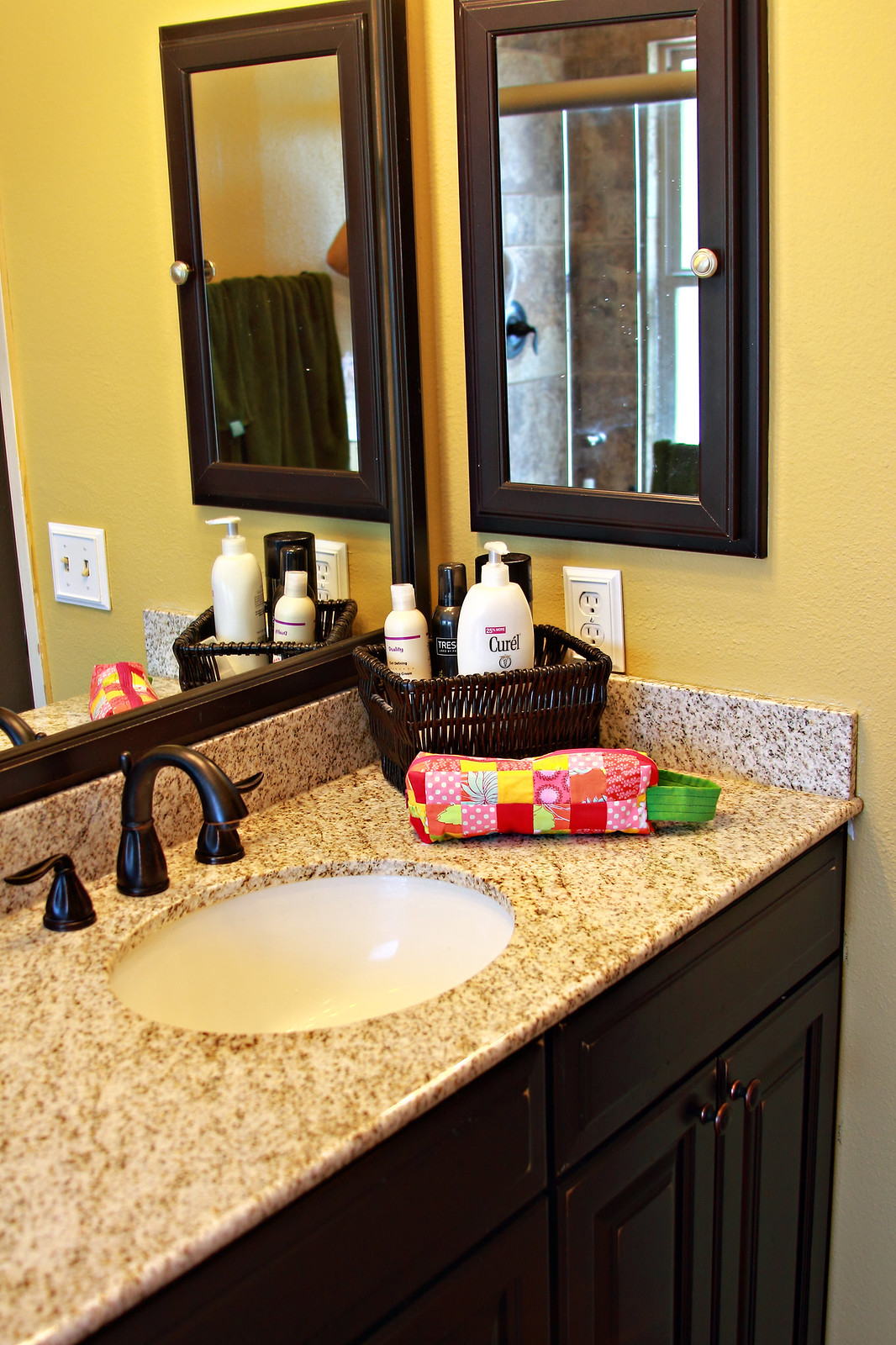This photograph captures a detailed view of a washroom. At the center of the image is a dark brown cabinet adorned with matching brown handles. A cream-colored countertop with brown speckles rests atop the cabinet, featuring a pristine white sink equipped with sleek black faucets.

On the countertop, there's a checkered bag in shades of pink and red, accented with a green handle. To the side, a brown basket sits in the corner, containing two black bottles and two white bottles, one of which is a lotion dispenser with a pump.

A large mirror with a black border hangs above the countertop, reflecting the entire scene. The washroom walls are painted a warm yellowish hue. Adjacent to the cabinet, another mirror is visible; this one has a door and a small handle.